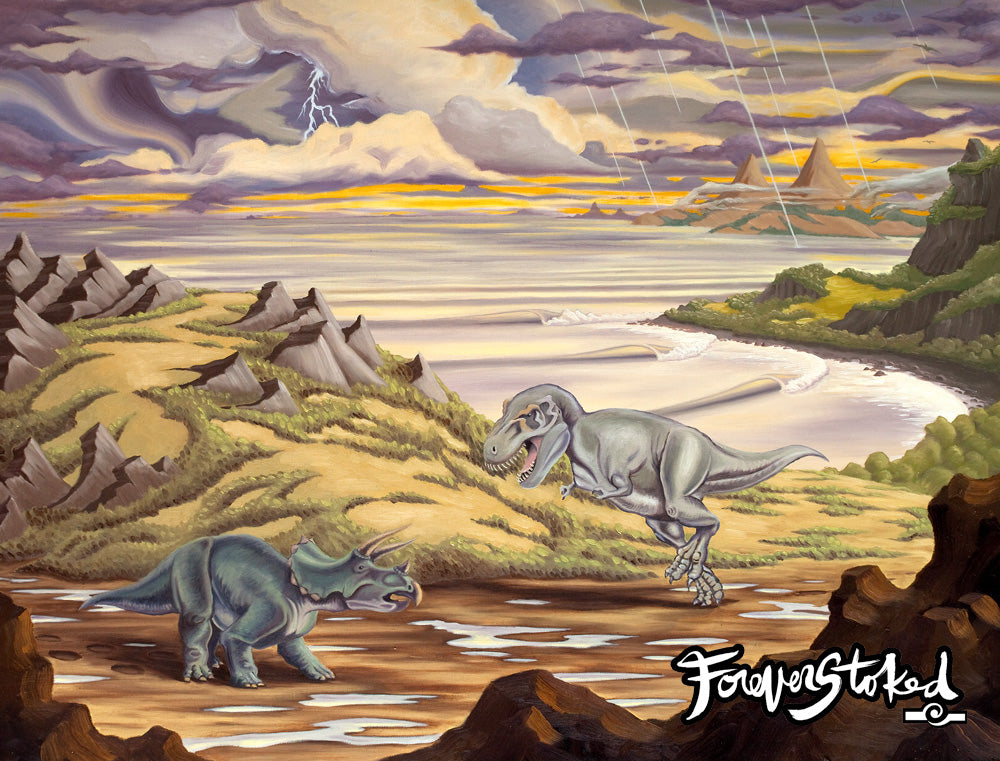The image is a detailed artistic depiction, possibly a computer simulation or painting, of a dramatic prehistoric scene featuring dinosaurs. In the foreground, on the lower left, a calm Triceratops with two prominent horns and a rhino-like body stands on sandy-colored land scattered with puddles. On the lower right, a fierce Tyrannosaurus rex rears up on its powerful hind legs, tiny front limbs poised, and its mouth agape, revealing rows of sharp teeth, seemingly charging towards the Triceratops. This dynamic interaction suggests an impending confrontation.

Behind the dinosaurs, a hill with jagged rock formations extends into distant mountains, beyond which lies a shimmering body of water with waves lapping at the shore. The sky above is filled with tumultuous dark clouds, pierced by dramatic lightning bolts and what appear to be streaking meteorites or rays of light, adding to the sense of tension and chaos. In the lower right corner of the image, the phrase "Forever Stoked" is elegantly inscribed in a stylized font, serving as a watermark for the piece.